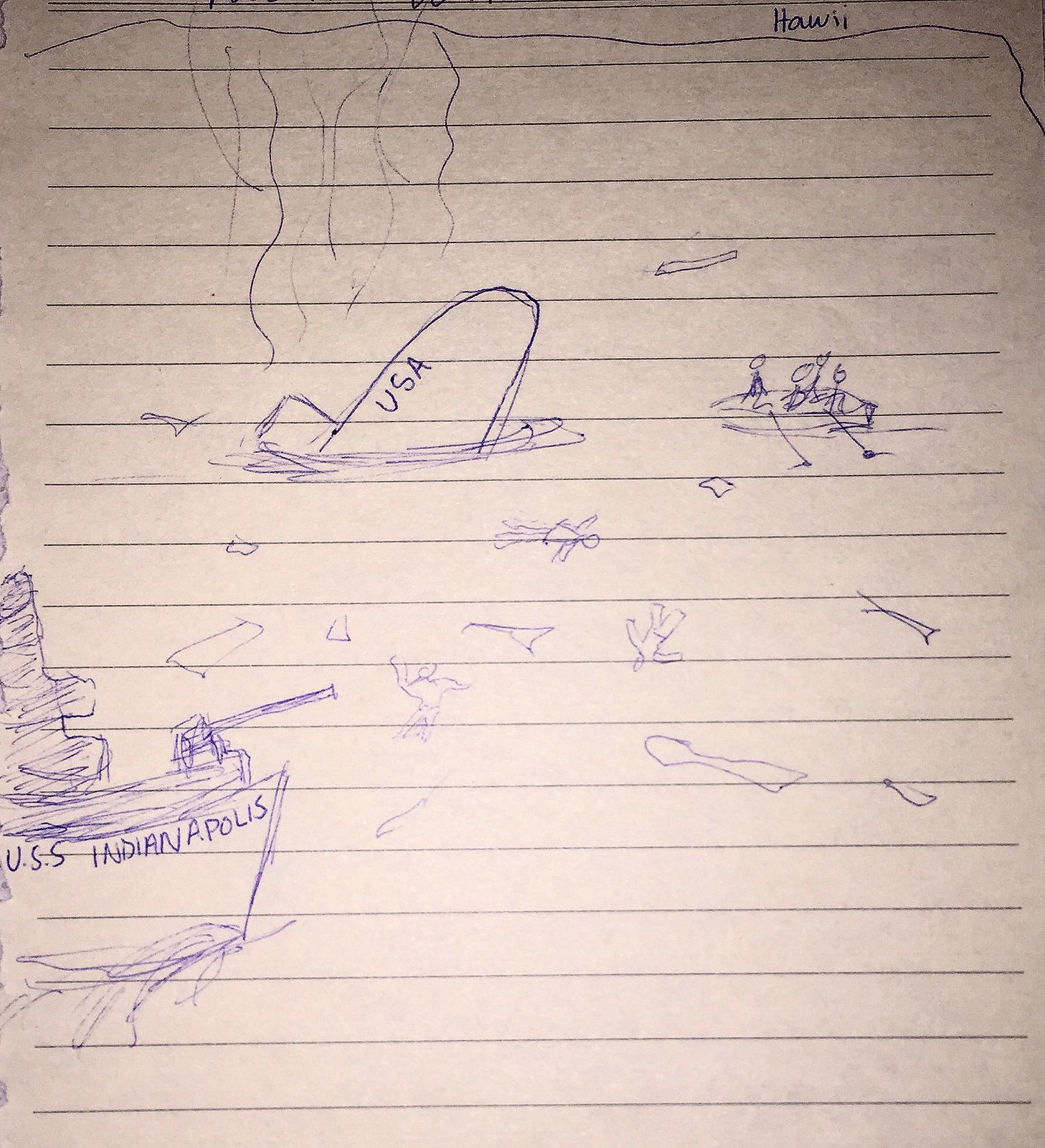The image, a detailed ocean scene drawn in blue ink on lined paper, prominently features a chaotic naval encounter. At the center, a sinking submarine labeled "USA" is half-submerged and in flames, surrounded by debris and many faceless figures floating in the water, suggesting a scene of distress. Four individuals are shown rowing away in a lifeboat with two oars, adding to the sense of urgency and desperation. In the lower left corner, a larger ship named USS Indianapolis is visible, armed with a cannon at its front. Above the turmoil, the word "Hawaii" is written, though misspelled as "H-A-W-I-I," encapsulating the dramatic maritime disaster unfolding below.